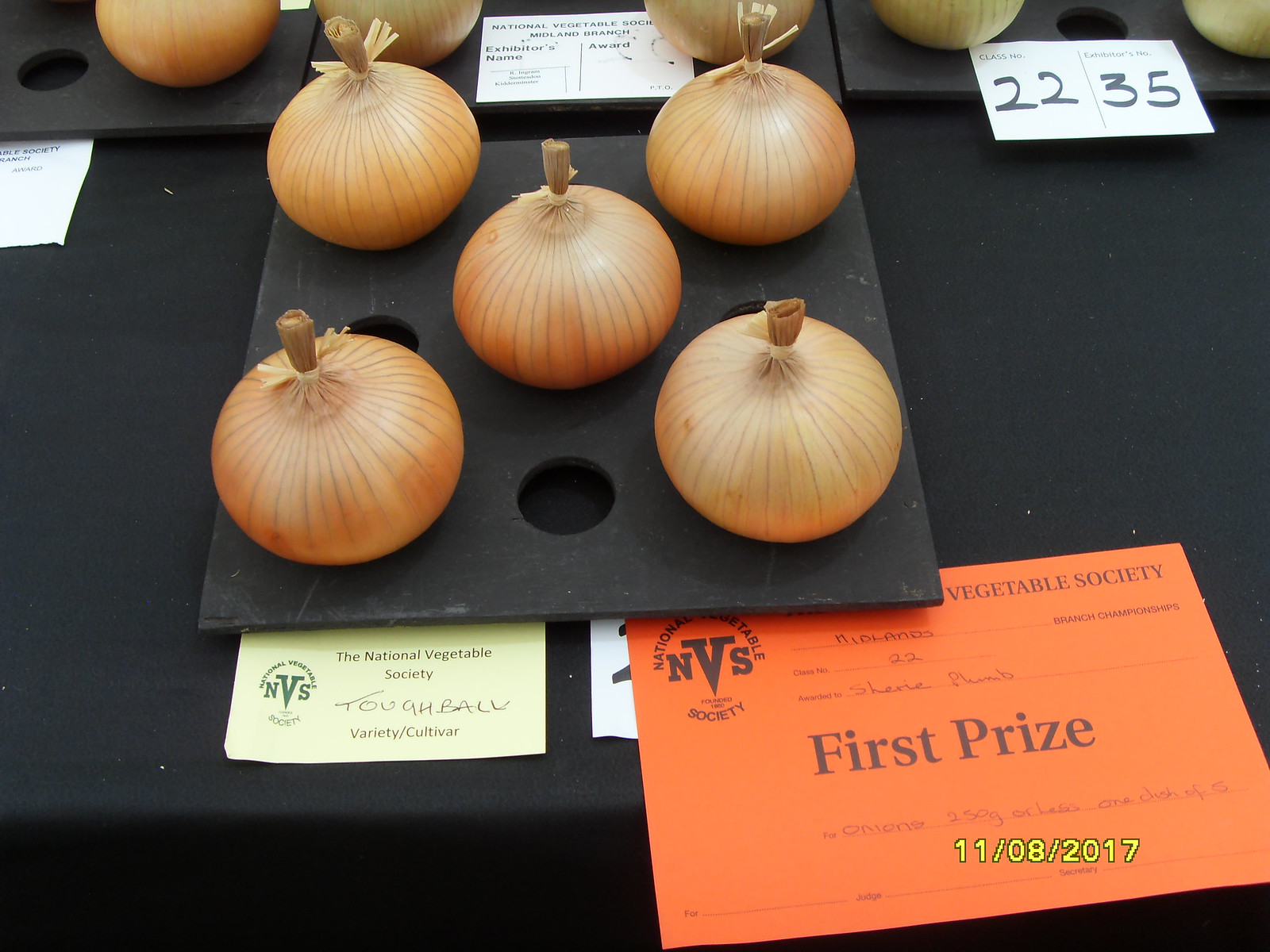This detailed caption describes an award-winning display of onions featured on a black-clothed table:

"The image shows a display of pristine onions arranged on a perforated platform, resembling the five-dot pattern on dice, with five onions placed perfectly in the center. The table, adorned with a black tablecloth, holds multiple trays featuring more onions, partially visible in the background. Each onion's outer peeling is fully intact, showcasing their flawless quality. A yellow sticker beneath the central tray reads 'National Vegetable Society' with the handwritten note 'Toughball,' and 'Variety/Cultivar' along with the MVS logo. An orange certificate indicating 'MVS' and 'first prize' is prominently displayed, awarded to Sherry Plumb for class number 22, as part of the Midland Branch championship. The award date is noted as 11-08-2017. In the top right corner of the image, a paper marked 'class number 22, SBTOS number 35' is visible, further emphasizing the recognition and achievement. White postcards or papers, possibly indicating further details, are seen on the trays in the background, one prominently displaying '2235'."